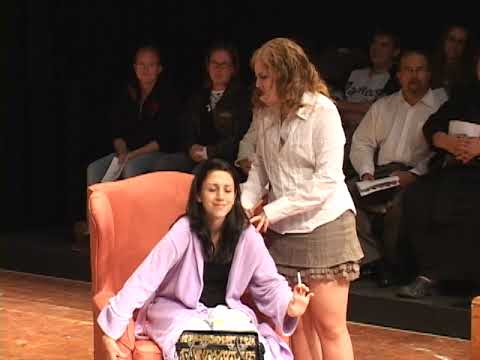In this real-world photograph, a central stage showcases two women in focus. One woman sits in a peach-colored recliner at the center of the platform, dressed in a light purple robe over a black shirt. She has long black hair and is holding a cigarette in her right hand, with a leopard print purse at her feet. Leaning forward with her eyes closed, she smiles while another woman stands beside her. The standing woman, who has long blonde hair, wears a white long-sleeve button-up shirt and a short gray skirt. Her hands rest gently on the seated woman's shoulders. Behind them, an audience attentively watches, some holding programs, seated in rows on the right and left of the stage. The floor beneath them is brown. The entire scene suggests a theatrical performance, with the two women likely being the central characters.